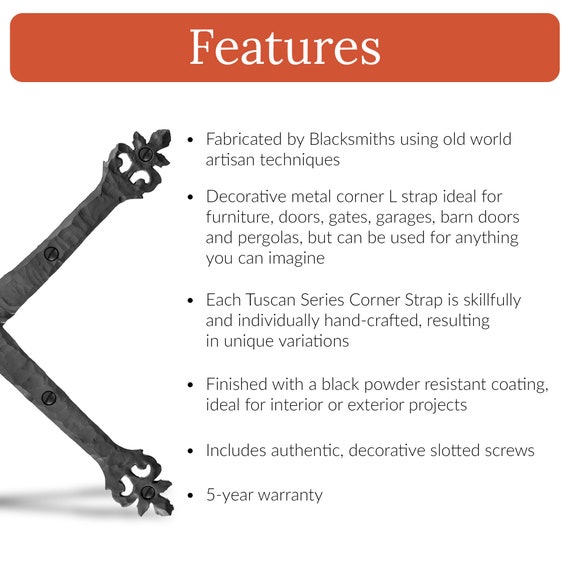The image features a PowerPoint slide detailing a product, specifically decorative metal corner L-straps. The top section includes a prominent big red banner with a bold white title that reads "Features." Below the title, the details are listed in smaller black text with bullet points. These bullet points elaborate that the L-straps are fabricated by blacksmiths using old-world artisan techniques and are ideal for a variety of applications including furniture, doors, gates, garages, barn doors, and pergolas, although they can be used for a wide range of other purposes. Each piece in the Tuscan series is skillfully and individually handcrafted, resulting in unique variations. The straps are finished with a black powder-resistant coating making them suitable for both interior and exterior projects. They also come with authentic decorative slotted screws and include a five-year warranty. Additionally, the image shows a picture of the metal L-strap, characterized by its dark gray color and the ornate ends, accompanied by visible screws.